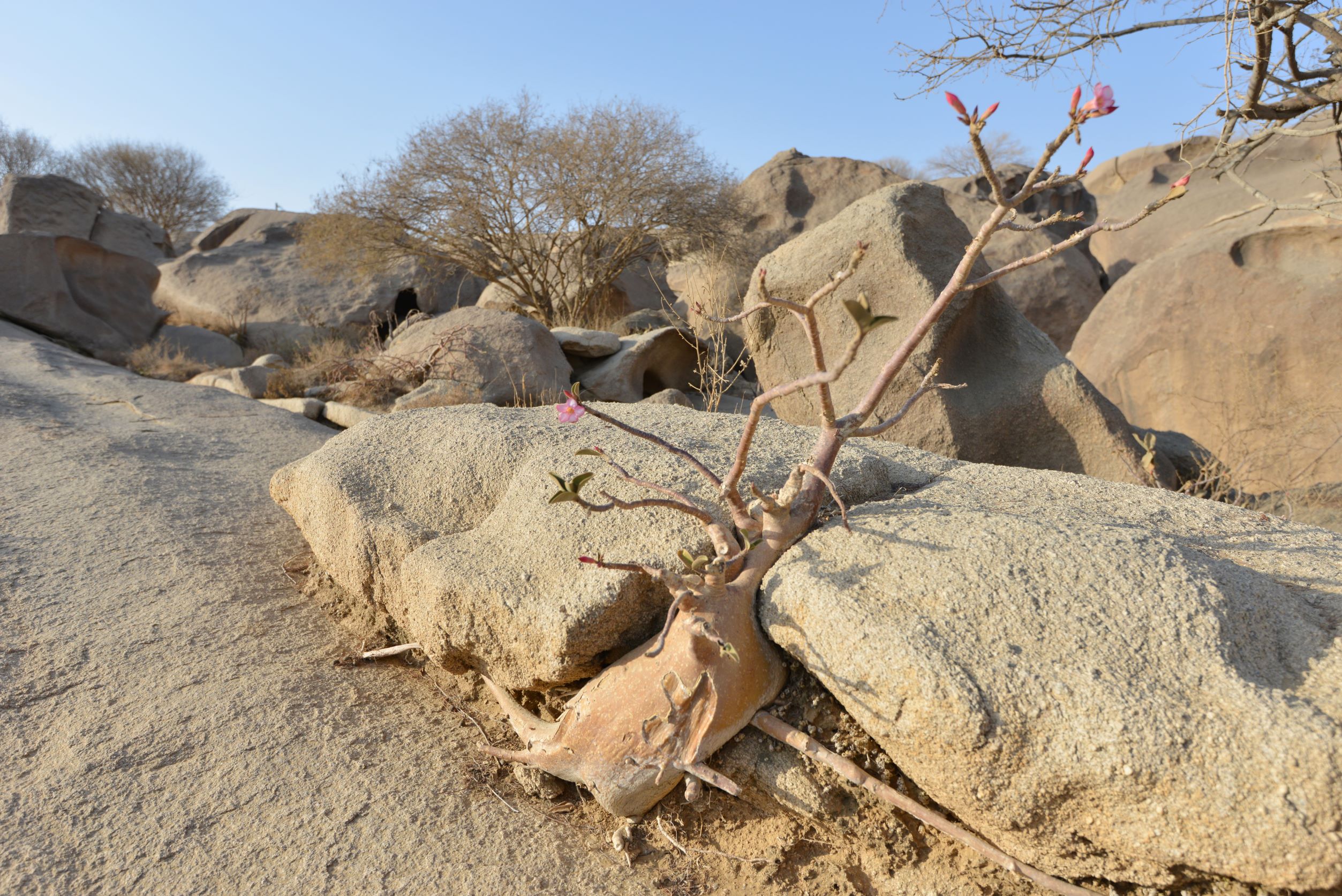The color photograph captures an arid desert landscape, dominated by large, weathered, sandstone-like boulders situated on a sandy terrain. Prominently nestled between two of these tan rocks is an intriguing plant, which appears almost like it's squeezing through a narrow gap. This plant features a thick base and numerous branches reaching skyward. Some branches are adorned with small, bright pink flowers at their tips, while others bear vibrant green leaves. In the background, scrubby trees and large bushes are sparsely scattered, and a clear blue sky stretches above, enhancing the desolate yet captivating beauty of the scene. The absence of people, animals, and man-made structures highlights the raw, untouched nature of this remote, arid setting, reminiscent of the outback of Australia or the most arid regions of California.